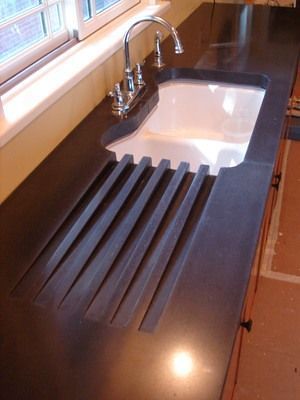A detailed photo captures the scene of a kitchen sink and counter from a vantage point at the end of the counter, looking along its length towards the sink. The sink, located in the far background, is a double-section white tub with two separate basins. The faucet features two knobs for temperature control and a prominent round, half-loop spout. Adjacent to the faucet on the right side, there is a detachable hose.

In front of the sink, a window with horizontal blinds and a sliding panel allows for natural light. To the left of the sink, a sloped drying rack, designed to channel excess water back into the sink, holds dishes for drying. The countertop itself is sleek black stone, contrasting nicely with the brown cupboards below, which are accented with black knobs. On the floor in the background, a piece of white tape is visible, adding a mundane but authentic touch to the everyday kitchen setting.